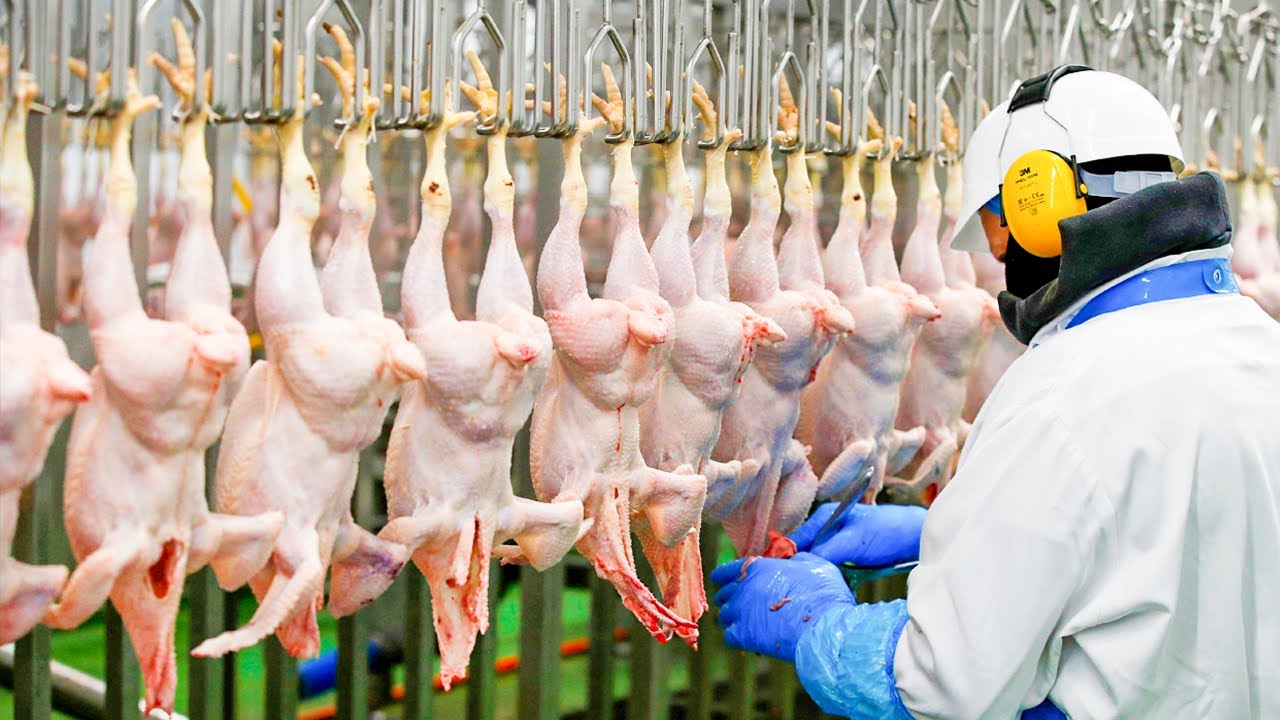The image depicts a silver metal processing machine adorned with dozens of defeathered, headless chickens that are suspended by their feet. A man is seen working with the machinery, clad in meticulous safety gear including a white helmet, yellow ear protection with small antennas, a black face mask, a white protective suit, a blue apron, and blue gloves. At the bottom of the scene, a fence is visible, beyond which lies a patch of grass, a red hose, and several blue objects scattered on the ground.